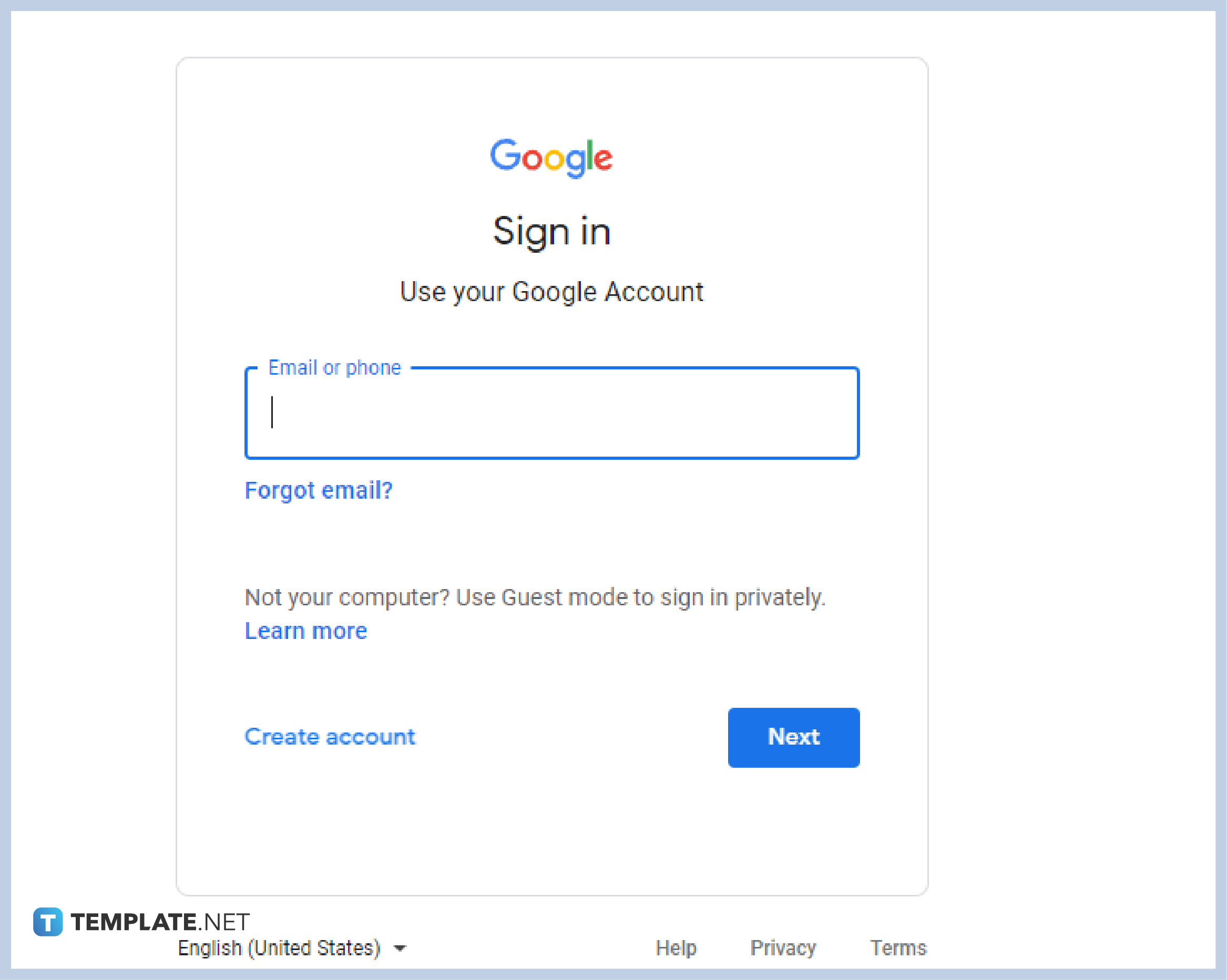The image depicts the Google account sign-in page with a clean and simple design. The page features a centrally aligned, gray-outlined rectangle against a white background. Surrounding this central area is a light blue border enhancing the page's structure.

At the top of the gray box, the word "Google" is prominently displayed, followed by the prompt "Sign in." Below this, the text "Use your Google Account" instructs users on what to do. A thin blue text box labeled "Email or phone" invites users to input their login credentials. Below this field is a link that says "Forgot email?" offering assistance for users who have misplaced their login information. 

Further down the page, there is a note saying, "Not your computer? Use Guest mode to sign in privately." A "Learn more" link in blue provides additional information. Moving lower, the page presents more white space leading to a two-option interface: on the left, a blue link labeled "Create account," and on the right, a prominent blue button reading "Next."

At the very bottom left corner, a blue box with a "T" logo is displayed with the text "template.net." Adjacent to this is a drop-down menu for language selection, currently set to "English (United States)." To the right of the drop-down menu are three linked options: "Help," "Privacy," and "Terms."

These navigation and assistance options are positioned outside the central gray-outlined sign-in box, finishing the clean and user-friendly layout of the Google sign-in page.